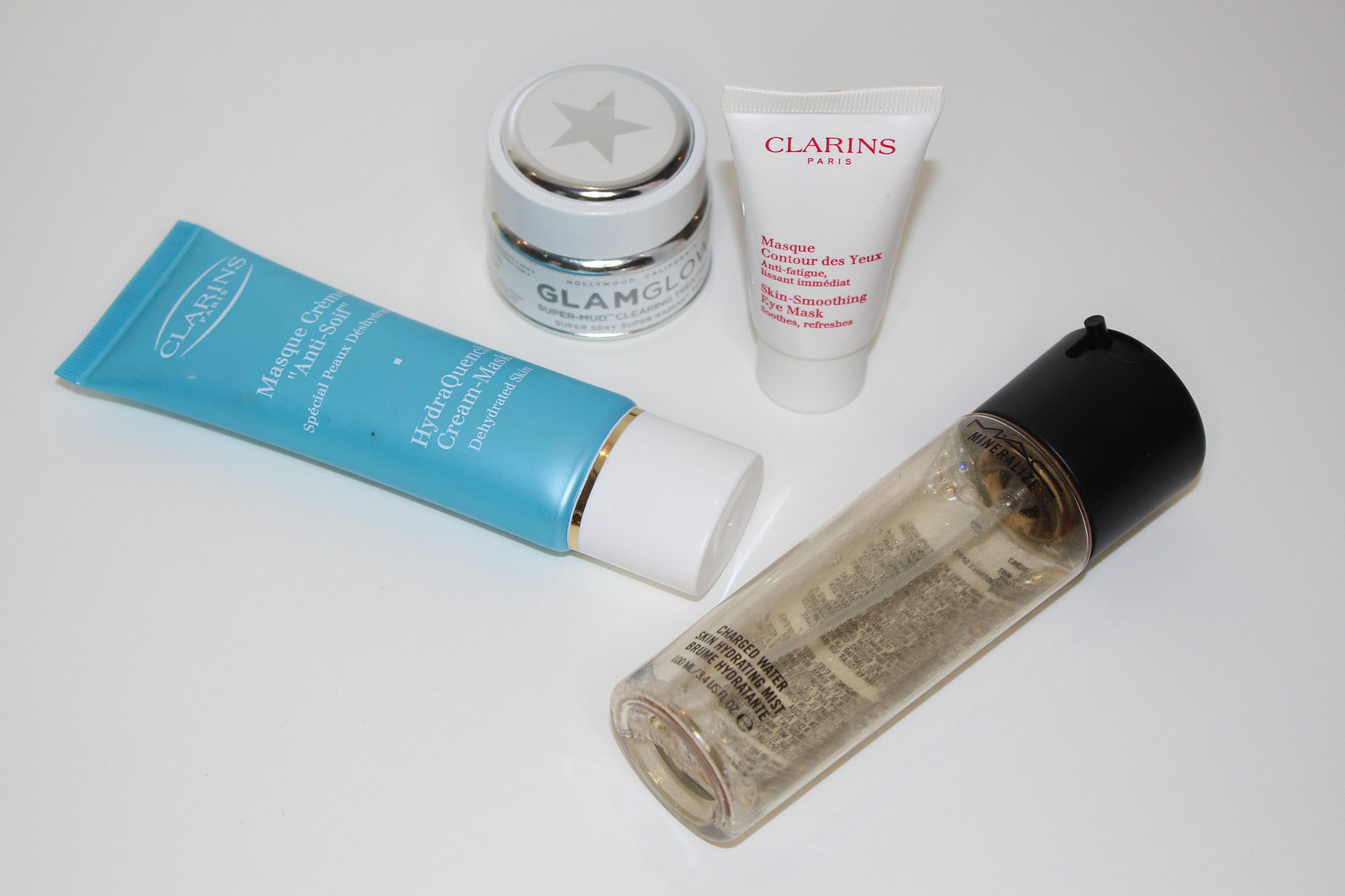In this visually captivating photograph of beauty products, the composition is artfully arranged against a pristine white background, resembling a serene bathroom countertop or an elegant showroom display. The image is landscape-oriented, with its width extending more than its height, providing ample space for the four featured items.

On the far left, a sleek blue tube of Clarins Masque Crème Anti-Soif Hydrating Cream Mask is prominently displayed. The tube is adorned with a sophisticated white lid, accentuated by a delicate gold band, lying horizontally for optimal display.

Next, moving rightward, the eye is drawn to a glamorous white and silver pot by GlamGlow, crowned with a light silver star etched on the top, exuding a sense of luxury and elegance.

Standing tall and proud in the lineup, the third item is a shorter tube, Clarins Paris Masque Contour des Yeux, an anti-fatigue, immediate skin-smoothing eye mask, designed to invigorate and refresh tired eyes.

The final product lies horizontally on the right side of the composition, featuring an amber-colored liquid encased in a sleek tube. Though not fully legible, the tube hints at the name "Mineralité" beneath the black lid and is identified as Charged Water, Skin Hydrating Mist (Brume Hydratante).

This collection showcases a harmonious blend of hydrating and rejuvenating beauty products, meticulously arranged to highlight their unique attributes and luxurious designs.